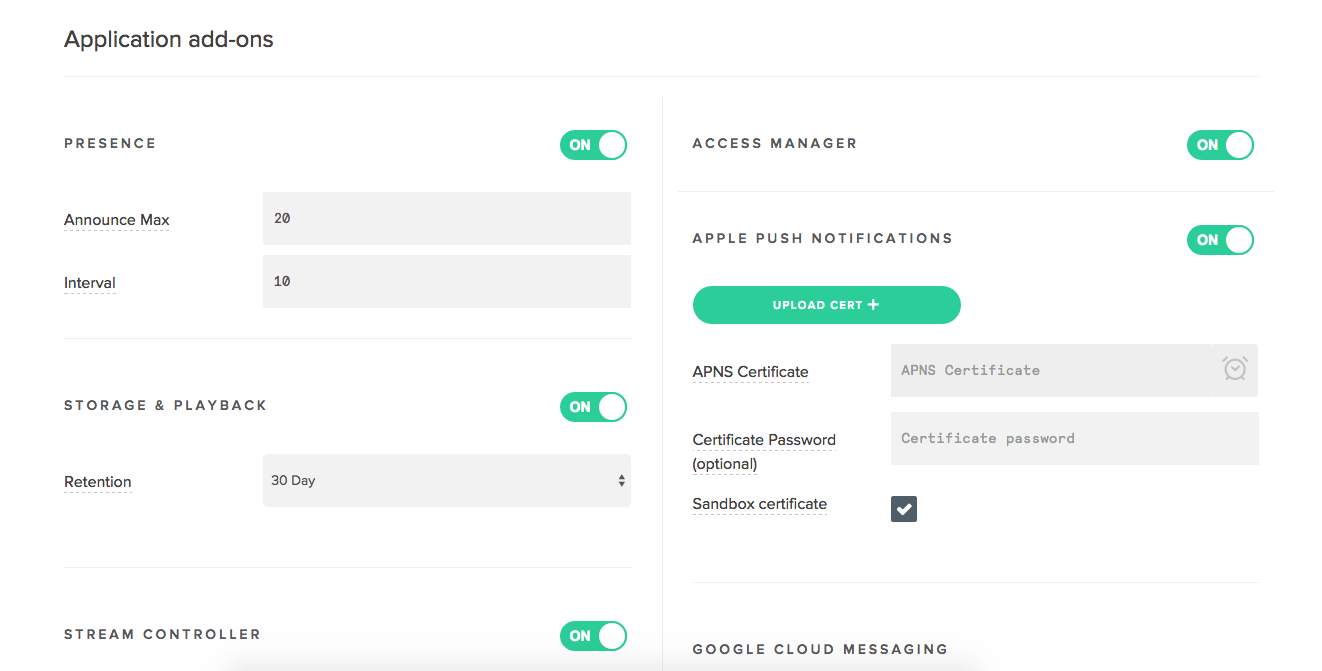In the photographic image of a web interface, at the top, we see the heading "Application and Add-ons" in black text. The section under it shows several configuration options. 

1. **Presence**: A green toggle switch is turned on.
2. **Announce Max**: There is a rectangular input box displaying the number 20.
3. **Interval**: Below "Announce Max," there is a gray input box showing the number 10.
4. **Storage and Playback**: This section has a green toggle switch turned on. Under it, labeled "Retention," the set value is 30 days, with adjustment arrows next to it.
5. **Stream Controller**: The toggle switch is green indicating it is turned on.
6. **Access Manager**: Also has a green toggle switched on.
7. **Apple Push Notifications**: This feature is toggled on in green.

Below these settings is a long green button labeled "Upload Cert +," with white text. The APNS (Apple Push Notification Service) Certificate section follows, featuring an alarm icon. There is also a field for "Certificate Password (Optional)," alongside options for a standard and sandbox certificate.